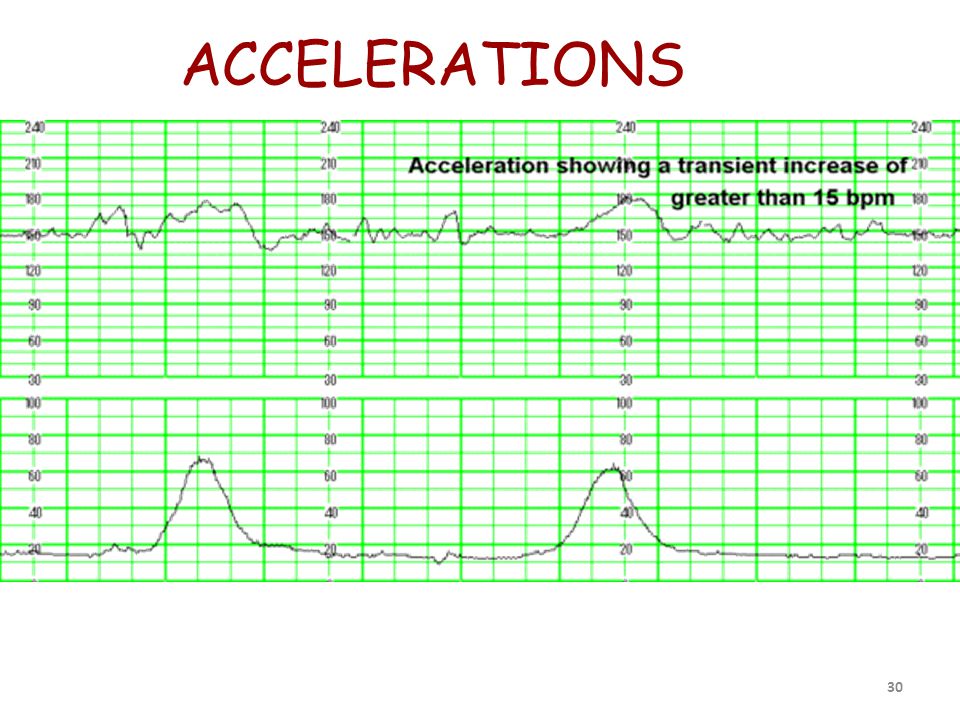The image depicts two detailed graphs, both with a distinct focus on heart rate accelerations, as indicated by the prominent red title "Accelerations" at the very top. The graphs are set against a bright, lime-green grid background. The upper graph is labeled with "Acceleration showing a transient increase of greater than 15 BPM" (beats per minute) and features a range of Y-axis values marked as 30, 60, 90, 120, 150, 180, 210, and 240. This graph displays a consistent, jagged pattern, characterized by numerous small peaks and troughs, suggesting continuous minor fluctuations in heart rate. 

The lower graph is marked with Y-axis values of 20, 40, 60, 80, and 100, and it shows a different pattern. Initially, the line remains low with minimal activity, then spikes sharply into a peak around 60 BPM before dropping back down into a deep valley near 20 BPM. This cycle repeats, showing only two prominent peaks interrupted by extended periods of low activity. Both graphs are organized in a square format with black numerical markers and line indicators, clearly delineated against the green grid to emphasize the fluctuations in heart rate accelerations.